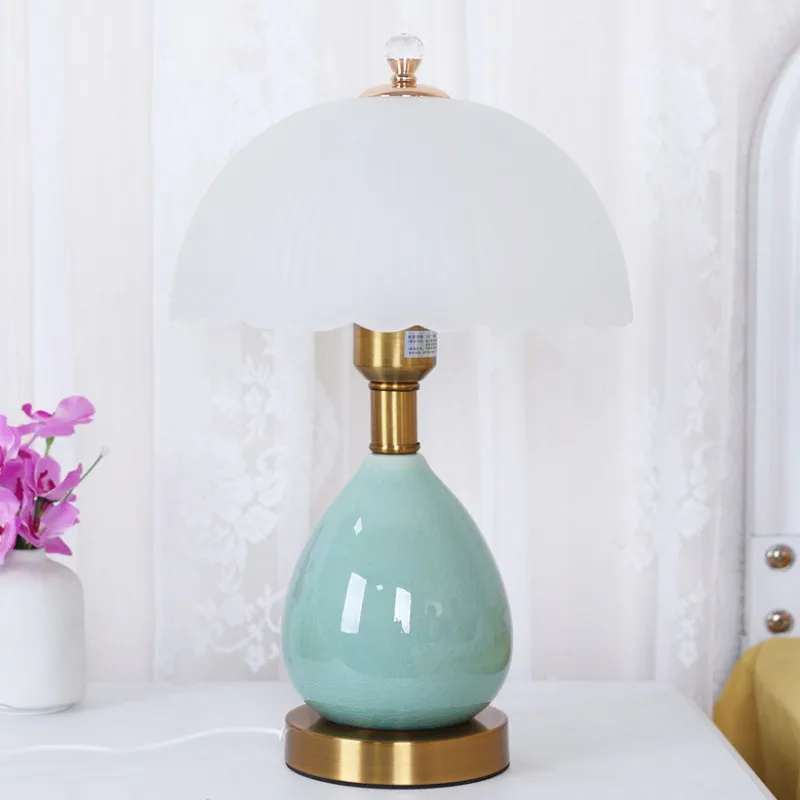This detailed image captures an elegant, luxurious lamp with a glossy, teardrop-shaped body in a soft pastel blue, made of glass. Its base and neck are a warm bronze color, creating a rich contrast with the pale bluish-green hue of the body. The lamp has a white, half-sphere lampshade adorned with subtle ridges along the bottom, giving it a refined look. This lamp is positioned on a pristine white tabletop. To its left sits a circular white vase filled with vibrant pink and purple flowers. The backdrop reveals sheer white curtains with delicate floral patterns. In the lamp's reflection, two windows suggest an indoor setting. Off to the right, there's a faint outline of a mirror on the wall, adding depth to the scene.